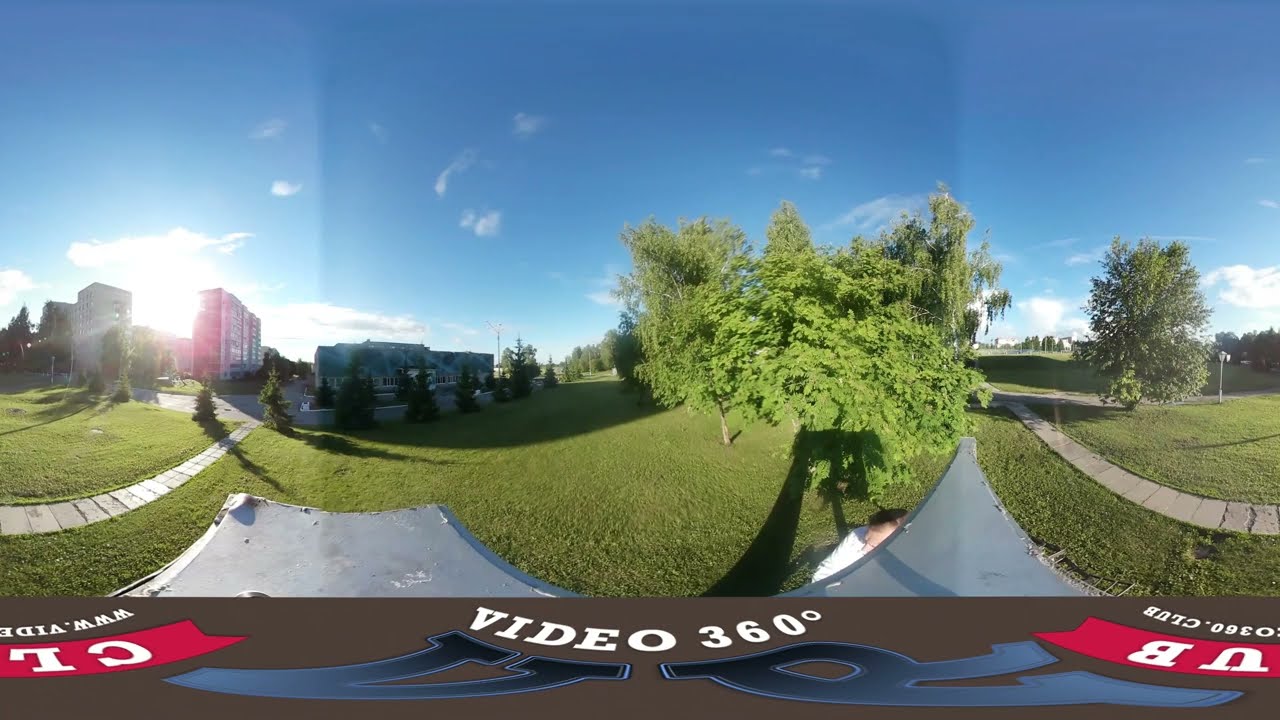The image depicts a horizontal and rectangular city park with neatly mown green grass. The park features a few scattered trees and is bordered by gray concrete sidewalks on both the left and right sides. In the background, there are taller buildings on the left, partially surrounded by trees, and several shorter trees line the right side. Above the horizon, a blue sky with a few clouds is visible. The bottom of the image includes a banner with "Video 360" written in white text on a black stripe, and to the right, large blue letters "V" and "R" are displayed. The image appears to be a screenshot from a video, potentially from an unusual camera angle, possibly giving a rounded perspective.